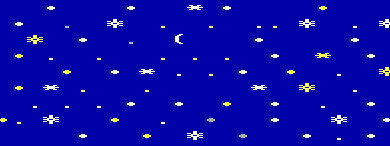This image is a digital rendering of a slim, dark blue rectangular background, reminiscent of a deep navy or deep-sea hue. Small, pixelated white and yellow elements are scattered throughout, resembling a nighttime sky. The pattern includes white crescent moons, various white and yellow asterisks that emulate either stars or snowflakes, and numerous small dots of varying sizes. While some dots are slightly larger, they all contribute to the abstract, yet recognizable depiction of a starry night. One prominent crescent moon sits slightly left of center, surrounded by more white stars than yellow. The design is not symmetrical, lending it a random, organic feel, much like a gift wrapping paper or a whimsical take on the night sky.